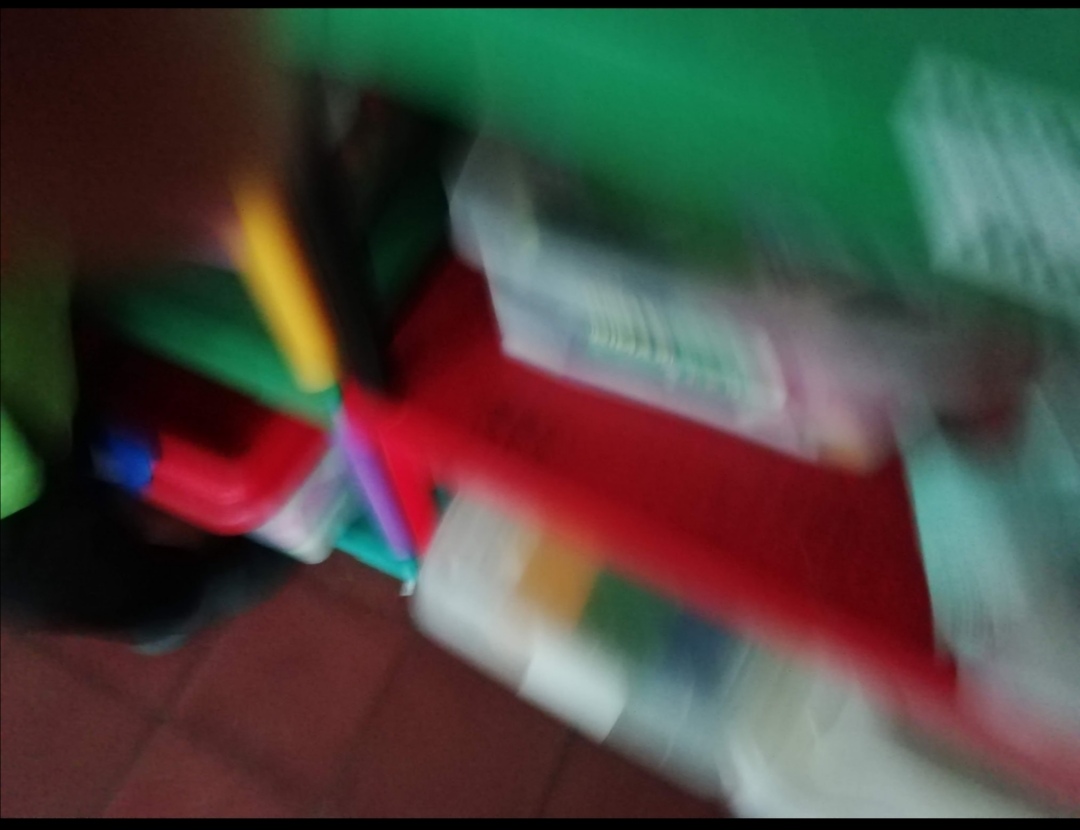A blurry image captures a downward view of colorful plastic shelves filled with clear plastic tubs. In the bottom left corner, the ground is covered with reddish square ceramic tiles separated by brown grout lines. The top left of the image shows a blurred object, possibly a finger. The shelves, vibrant in colors such as red, green, and yellow, house several plastic tubs, including one on the lower left shelf with a red and blue lid. Due to motion blur, the entire image, especially the white containers, appears somewhat smeared, suggesting that the camera was moving downwards and to the right when the photo was taken.